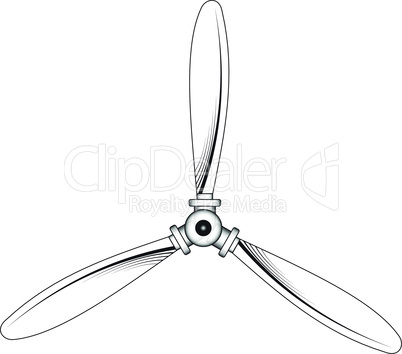The image depicts a white background with a drawn illustration of a three-bladed propeller. Each blade is white with a distinct black outline. The configuration displays one blade positioned directly at the top center, while the other two blades extend outwards to the left and right, creating a layout similar to a peace sign when circumscribed by an imaginary circle. The central hub of the propeller is marked by a black dot, suggesting a circular centerpiece with some shading that adds depth to the drawing. Over the propeller, there is a nearly transparent watermark that reads "Clip Dealer Royalty Media" with an accompanying faint logo. The watermark is subtle, making it challenging to decipher against the detailed line drawing of the propeller. Additional small shapes around the blade connections, resembling screws or caps, further emphasize the mechanical nature of the object, which might suggest an aircraft propeller or a fan.